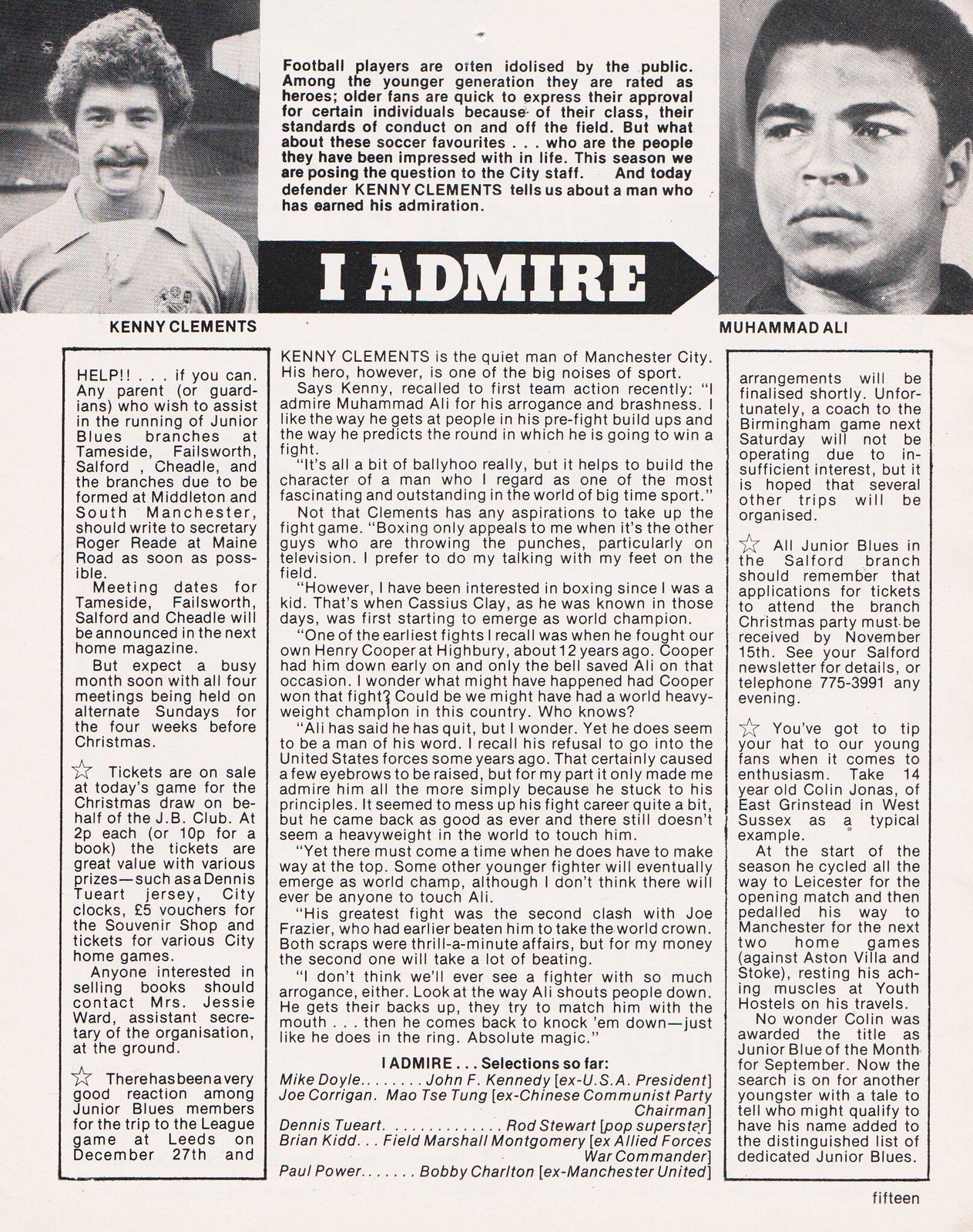This detailed image caption for the referenced article effectively merges elements from all three descriptions:

This is a black-and-white page from a Gameday magazine, specifically page 15, as indicated in the bottom right corner. The top left of the page features a profile photo of football player Kenny Clements, with his name below the image. Adjacent to this, there is an arrow pointing towards the top right, which encloses the text "I admire" in bold white letters. At the other end of the arrow is a profile photo of Muhammad Ali, also with his name below it, visually indicating that Kenny Clements admires Muhammad Ali. Above the arrow, a brief synopsis mentions that football players are often admired by the public and details what it takes to earn admiration. The article predominantly focuses on Kenny Clements, his career, and his admiration for Muhammad Ali. Additionally, at the bottom of the page, there is a section listing other sports figures and the people they admire, including Mike Doyle's admiration for John F. Kennedy, Paul Power for Bobby Chardon, and Dennis for Rod Stewart.